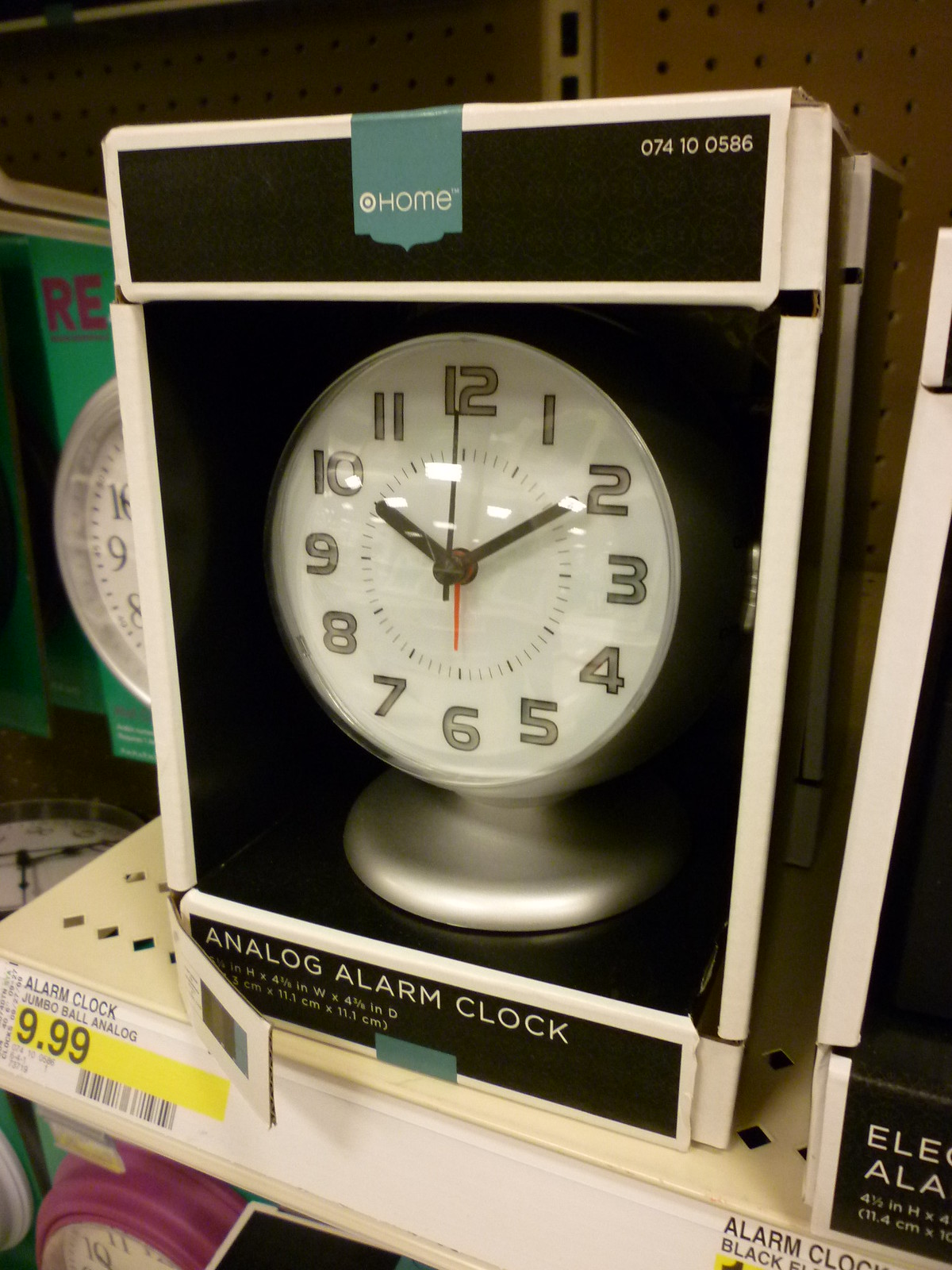This indoor photograph captures an analog alarm clock positioned on a store shelf, still nestled in its original packaging. The clock boasts a round, bubble-shaped plastic face encasing a white dial. Bold, clear gold numbers from 1 through 12 encircle the dial, which displays the time as 10:10, with the second hand precisely on the 12. The packaging prominently features the text "Analog Alarm Clock" at the bottom and "At Home" on the top. The shelf label beneath the clock indicates a price of $9.99. Adjacent to this clock, the edge of another clock peeks into the frame, and to the left, a partial view of yet another clock face with a distinctive green case can be seen.